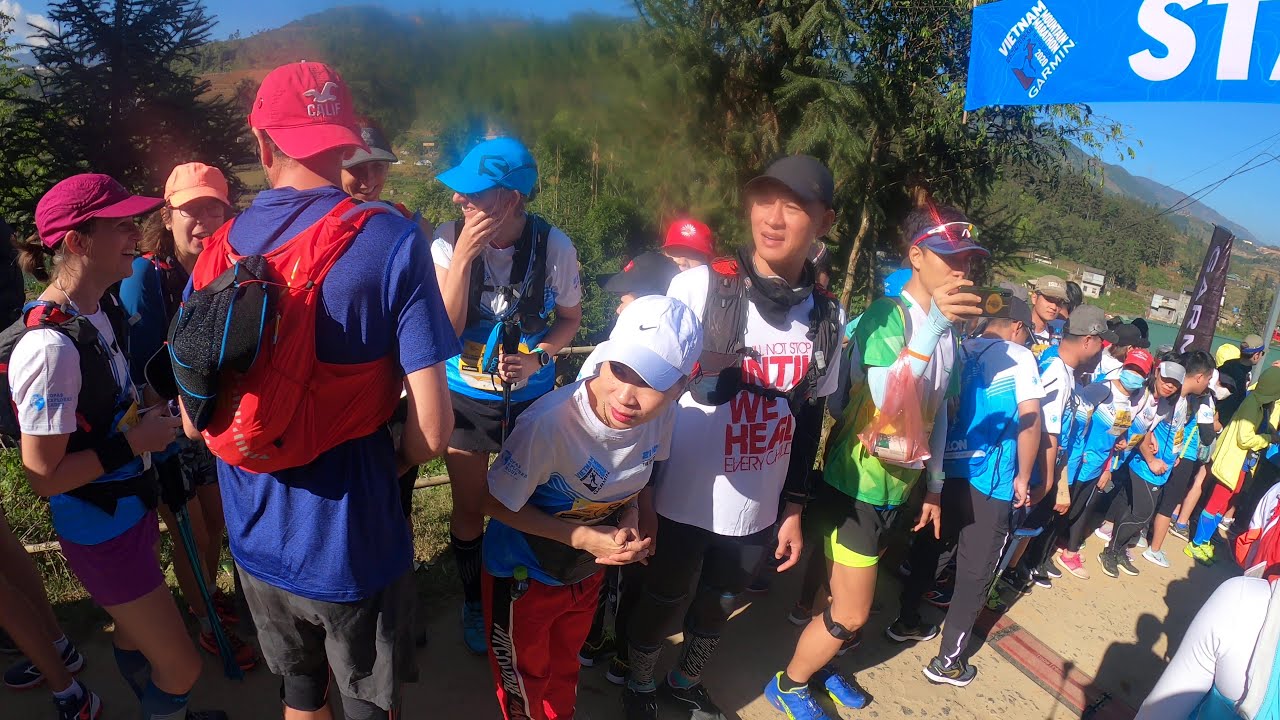This vibrant outdoor scene from Vietnam captures a large group of people, likely around 60 or more, gathered at the starting line of a trail event, possibly a hike. The participants are dressed in hiking or jogging attire, with most wearing hats and backpacks. The line of people extends horizontally, curving slightly downward to the right. Prominently displayed above them is a blue banner with white letters, partially readable as "Vietnam Garmin," possibly indicating sponsorship by the GPS manufacturer Garmin. The sign also includes letters "ST," suggesting it marks the starting line. The setting is picturesque, with a clear, sunny sky and a backdrop of green, hilly terrain covered in grass and trees, indicating a mountainous area. The participants stand on what appears to be a wooden deck or platform, with a serene environment featuring structures that suggest nearby homes and a small lake or pond.